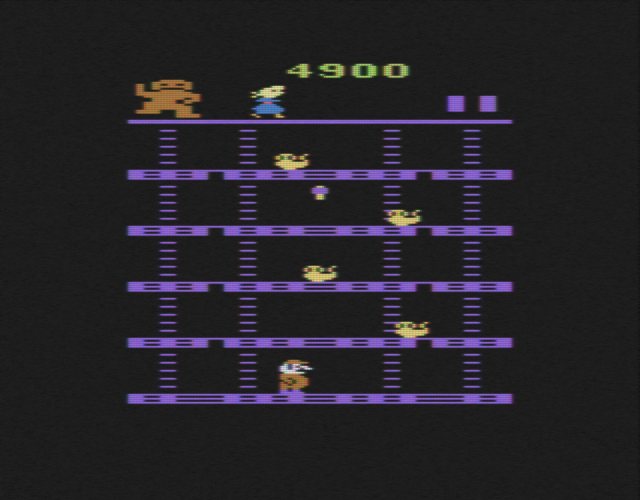The image is a still from an old video game reminiscent of a classic Atari 2600 or Nintendo game, featuring a dark black background with a series of horizontal, purple platforms. At the top, the game displays a score of 4900 and indicates two remaining lives in the upper right-hand corner with simple line symbols. These platforms are interconnected by dashes symbolizing ladders, with four ladders per level, giving players multiple paths for vertical movement. 

On the uppermost platform, there's a large orange figure, likely representing Donkey Kong, positioned in the corner, with a feminine character dressed in blue nearby, possibly held captive. The game's objective appears to involve the character Mario, depicted in brown attire at the bottom level, navigating upward through the five levels using the ladders. Players must avoid or jump over various obstacles, including yellow, snake-like creatures scattered across the levels. Additionally, several gold lamp-like objects can be seen on the platforms, which players might need to collect. This image captures the distinctive vintage video game aesthetic and strategic platform layout typical of early gaming.